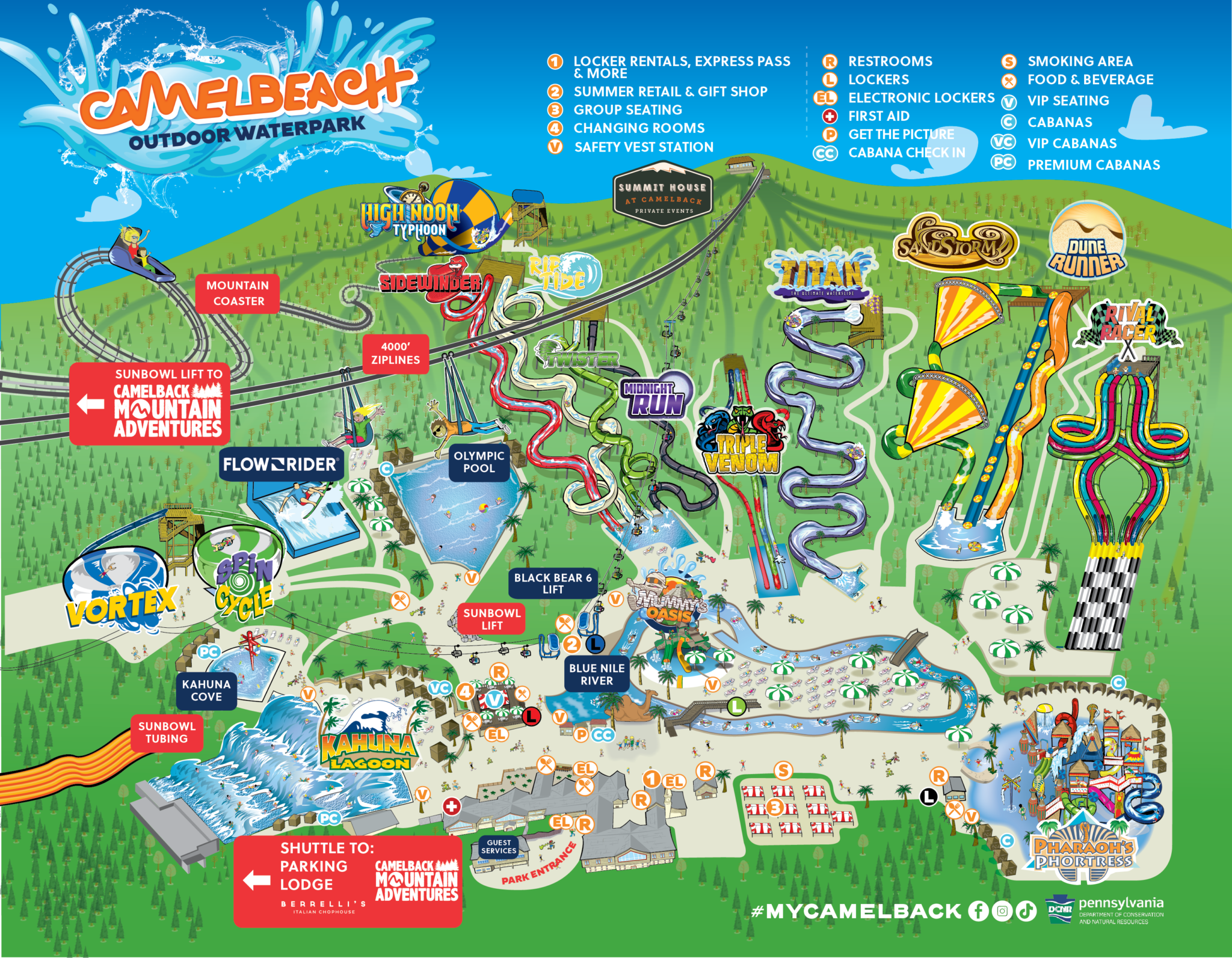The image is a detailed map of Camel Beach Outdoor Water Park, prominently titled in the top left corner. The map showcases various rides and attractions scattered across a colorful layout, with rides identified from left to right including High Noon Typhoon, Sidewinder, Summit House at Camelback, Titan, Sailstorm, Dune Runner, Midnight Run, and Kauna Lagoon. The map's color scheme features vibrant hues of green, blue, red, yellow, black, and white, highlighting different sections and themes of the park.

The amenities are clearly marked, showing areas for locker rentals, an Express Pass, a summer retail and gift shop, group seating, changing rooms, a safety vest station, restrooms, lockers, and electronic lockers. Other facilities include first aid, "get the picture" booths, cabana check-in, a smoking area, food and beverage stalls, VIP seating, VIP cabanas, and premium cabanas. The map has numbered labels for easy navigation, and a key for services and locations.

The park's layout suggests it is situated on a mountainous terrain, reflected in its green background and dotted with tree illustrations. At the bottom of the map, the hashtag #mycamelback is displayed, indicating the park's association with Camelback in Pennsylvania. This elaborate map provides a comprehensive view of all rides and amenities, making it easier for visitors to plan their experience.